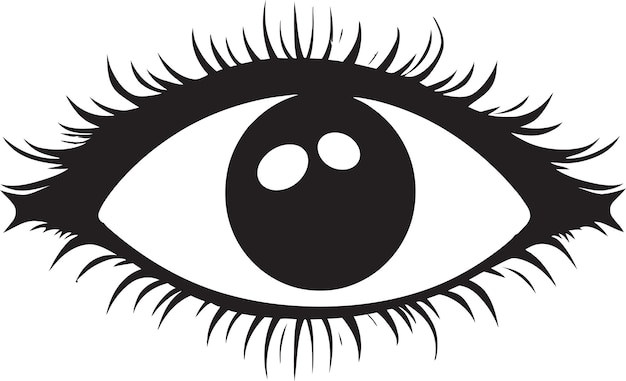This black-and-white artistic drawing depicts a detailed human eye on a white background. The eye's oval shape, reminiscent of a football, is defined by thick black lines, with the top lid showcasing heavier outlining compared to the bottom lid. The pupil, centered within the eye, is a solid black circle featuring two distinct white reflection highlights positioned at approximately the 10 o'clock and 12 o'clock angles, giving the eye a sparkling effect. Both the top and bottom lids are adorned with plentiful, thick eyelashes that curl outwards, the top lashes extending upward and the bottom lashes curling downward. The lashes fan out in various directions, creating a sense of depth and realism. The outer edges of the eye exhibit a concave curve, adding to the dynamic and somewhat stylized nature of the drawing. Overall, this illustration echoes a cartoonish yet detailed aesthetic, comparable to the animation style of "The Nightmare Before Christmas."